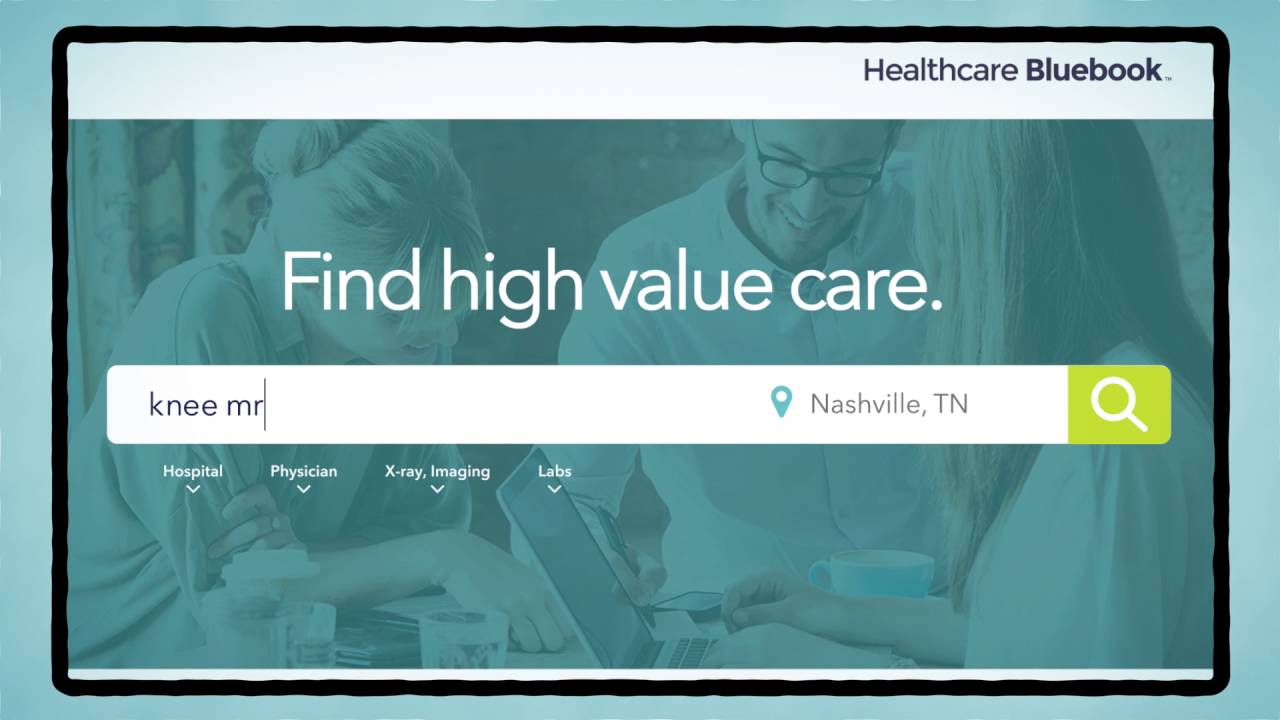This detailed caption provides an in-depth description of an apparent healthcare-related advertisement.

Screen capture of a healthcare advertisement. The central area features a white and blue square, with an inner black-outlined box in a pale blue hue. At the top, “Health Care Blue Book, TM” is prominently displayed in black text. Below that, in large white font, is the phrase “Find High Value Care.” Further down, there is a white search box containing the typed text “knee MR” in black, alongside a cursor icon. Adjacent to the search box is a teal location pin with “Nashville, Tennessee” written in gray. To the right, a green box with a white magnifying glass icon signifies a search function. Submenus listed below include categories for Hospital, Physician, X-ray, Imaging, and Labs, each accompanied by a down arrow.

In the background, a superimposed image shows a smiling woman with hair in a bun, wearing a ring and a rolled-up sleeved shirt, holding a coffee cup. Next to her is a smiling man with black glasses and a white shirt, a cellphone in front of him. Another woman, dressed in white and working on a laptop, is looking at the man. A coffee cup is also visible next to her. The background interaction suggests a casual, friendly atmosphere among the individuals.